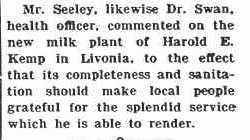The image depicts a small, grainy, rectangular excerpt that appears to have been scanned from an old newspaper or book. The background is predominantly white with a mottled grayish hue and occasional bluish light gray spots, giving it a vintage look. A prominent black line runs along the far left of the image, acting as a border. The centered paragraph, written in a small, slightly blurry, black font, reads: "Mr. Seeley, likewise Dr. Swan, Health Officer, commented on the new milk plant of Harold E. Kemp in Livonia to the effect that its completeness and sanitation should make local people grateful for the splendid service which he is able to render."